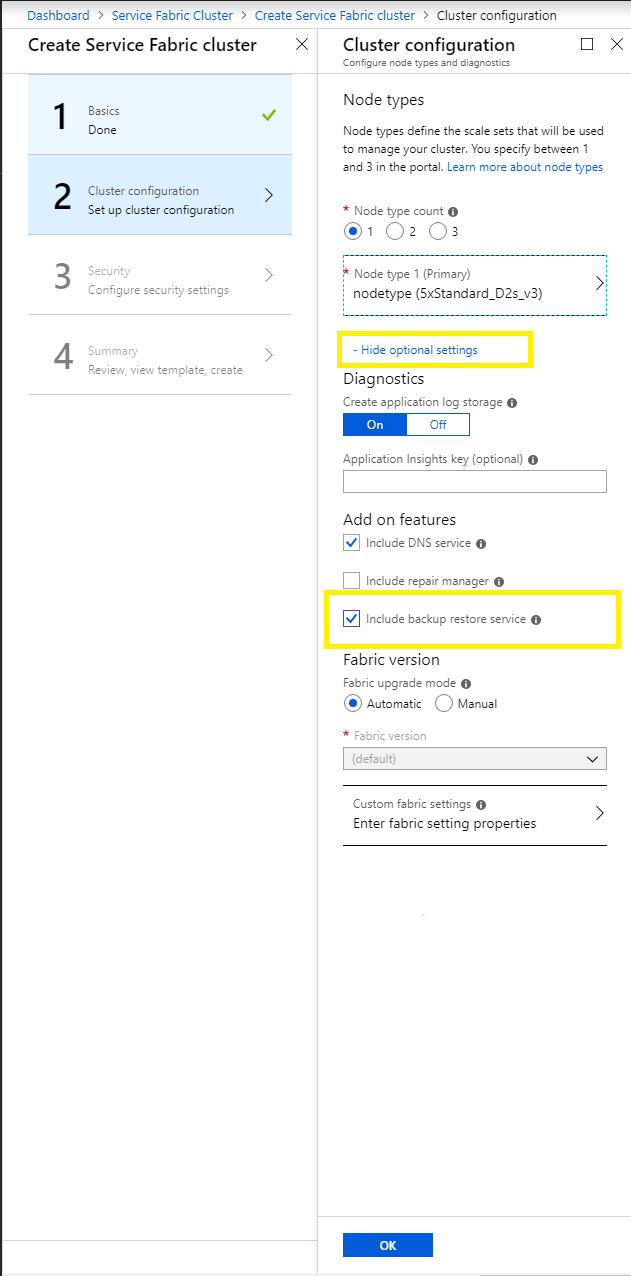### Descriptive Caption

**Dashboard View for Creating a Service Fabric Cluster: Detailed Configuration Breakdown**

The dashboard displays a step-by-step process for creating a Service Fabric Cluster. 

1. **Basices Section (Marked Done with Checkmark):** Basic configurations are already completed.
2. **Cluster Configuration Setup (Highlighted with Arrow):** 
   - **Node Types and Diagnostics Configuration:**
     - Users can specify node types, which are crucial for defining the scale sets to manage the cluster. The portal allows specifying between 1 and 3 node types. 
     - A red star indicates mandatory fields such as "Node Type Count," which lists:
       - 1 (Blue Dot)
       - 2 (White Circle)
       - 3 (White Circle)
     - The primary node type is marked with parentheses and indicates detailed specs: "5X Standard D2S V3."
     - Certain fields such as "Hide Optional Settings" are highlighted in yellow.
   - **Diagnostics Section:**
     - Users can enable or disable application log storage.
     - Option to add an Application Insights Key is available but optional.
   - **Add-on Features:**
     - Includes options such as DNS Service and a blank checkbox for the Repair Manager.
     - "Include Backup Restore Service" has a blue checkbox alongside a yellow highlight.
   - **Fabric Version Configuration:**
     - Users can toggle between Automatic and Manual modes for fabric version selection.
     - "Fabric Version" field is mandatory, indicated by a red star. Users can choose between "Default" or "Custom" from a dropdown menu.
   - **Fabric Settings:**
     - Includes an inner properties arrow for further configurations.

This meticulously detailed interface guides users through creating and configuring a Service Fabric Cluster effectively, ensuring all necessary settings are properly addressed.